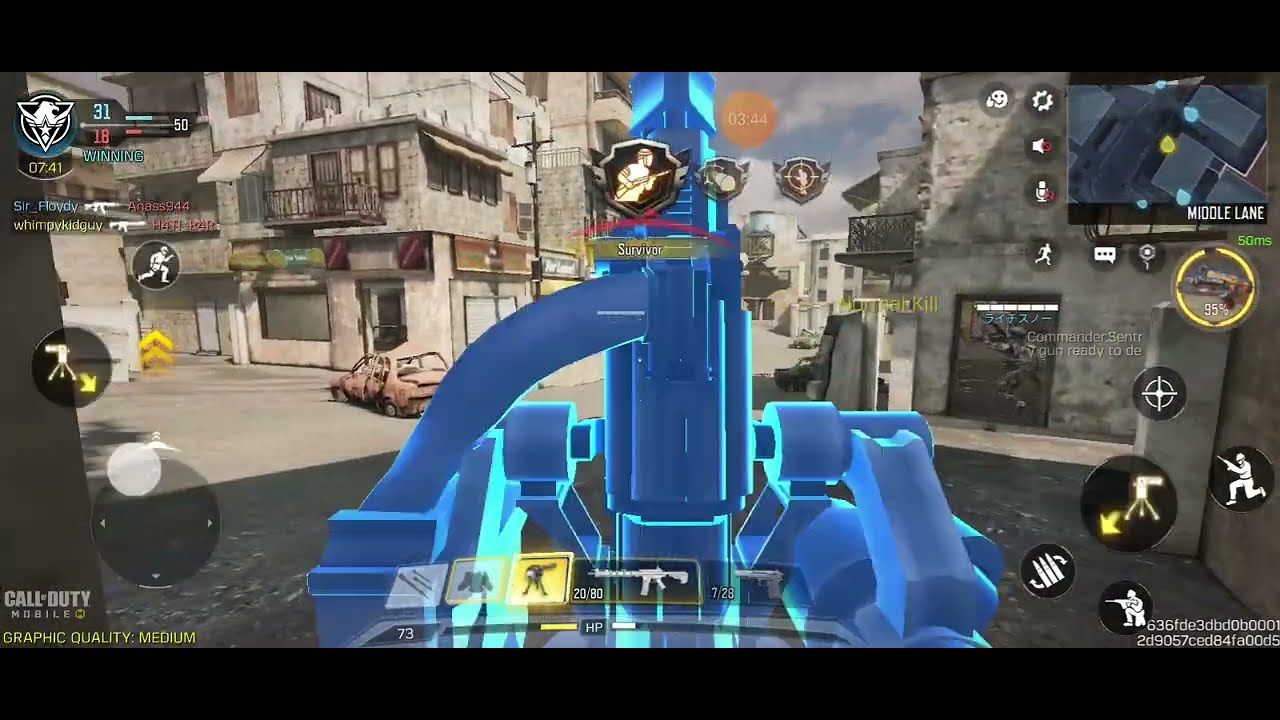The image is a detailed screenshot from the game Call of Duty Mobile, as indicated by the text in the bottom left corner stating "Call of Duty Mobile, Graphic Quality Medium." The scene is set in an urban environment, possibly a Middle Eastern city, characterized by multi-story gray buildings lining both sides of the street. Dominating the center of the image is a blue turret being placed by the player, which appears prominently in the foreground. Next to it, the interface shows that the player is holding a blue automatic assault rifle, pointed forward, with an ammunition count indicating 20 bullets left in the magazine and 80 in reserve.

In front of the gray building on the left side of the street, there's a noticeably damaged pink car. The image also features various game interface elements: buttons and health bars at the bottom, a map in the top right corner showing player locations, and game statistics on the left side detailing player kills. The colors seen in the screenshot include black, gray, white, blue, yellow, red, and orange, contributing to the immersive, action-packed atmosphere typical of a first-person shooter game.